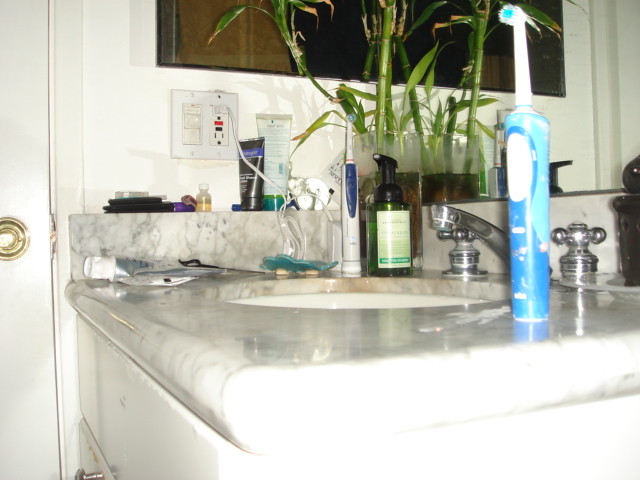The image depicts a bathroom scene. On the left-hand side, there's a door featuring a gold handle. The walls are painted in a greenish cream color. Adjacent to the door is a plate with a light socket and plug-ins. Moving towards the center, the wall transitions in color; it is brown on the far left, then black, and finally a gray-black on the right-hand side. In front of the wall, there's a potted plant, beside which are two tubes - one black and the other light green with a dark green cap. The sink's counter has a metallic silver finish that gradually blends into white. On the counter, there is an item with a blue-green hue, possibly a container. Additionally, there appears to be a toothbrush and a pump container with a black top and green bottom, featuring a light green label and a darker green rectangle at the bottom. Another toothbrush, light blue, dark blue, and white, is positioned in the foreground on the right-hand side.